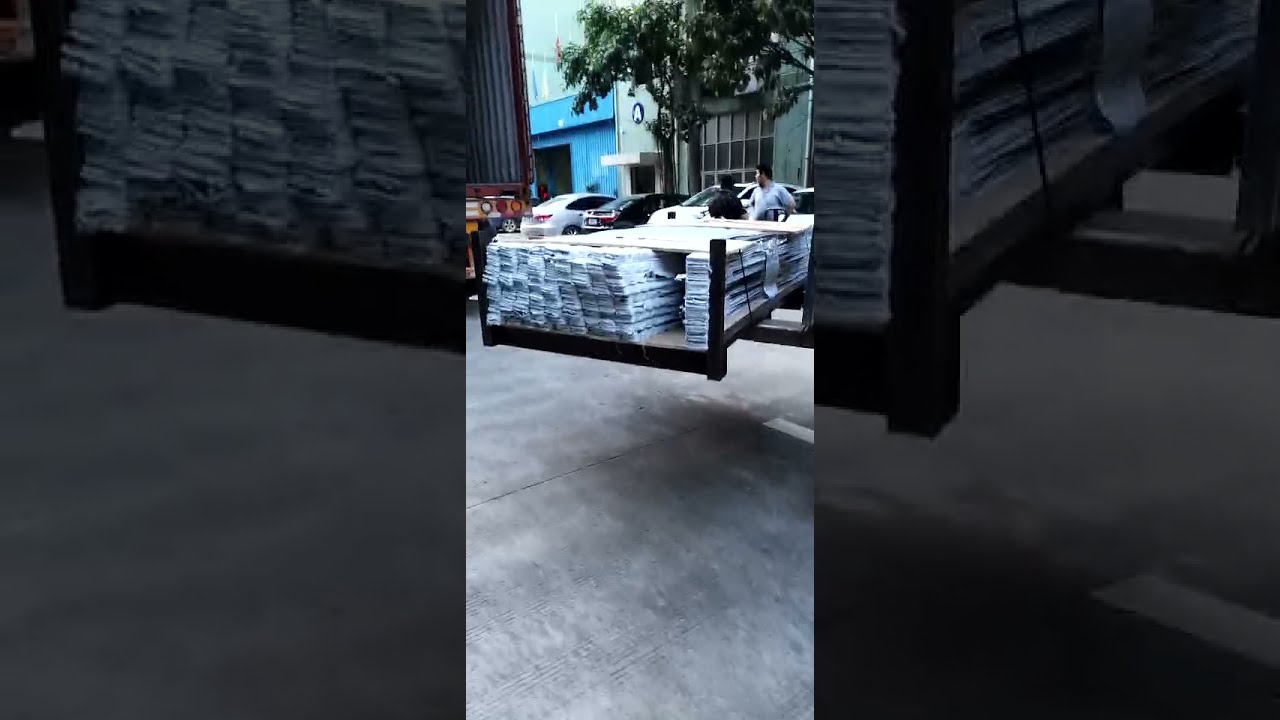In a vertically oriented cell phone picture, an intriguing pallet of goods is seen floating off the ground in a parking lot, with indistinct echoes of the image forming a faded background. The pallet, which seems to be loaded with bags of fertilizer or long, thin planks of wood wrapped in shrink wrap plastic, reveals the unusual sight of being elevated by the metal arms of a forklift seen to the right. Surrounding this central subject, the backdrop includes a mix of cars parked around what appears to be a blue and white building, reminiscent of either a factory or a car dealership. The building features large windows, a white entrance topped with a blue circle and the letter “A,” and a tree situated in front. A large loading truck is noticeable to the left. Additionally, inset within the picture is a smaller highlighted image, showcasing a line of cars and two indistinct figures in conversation in front of the dealership.